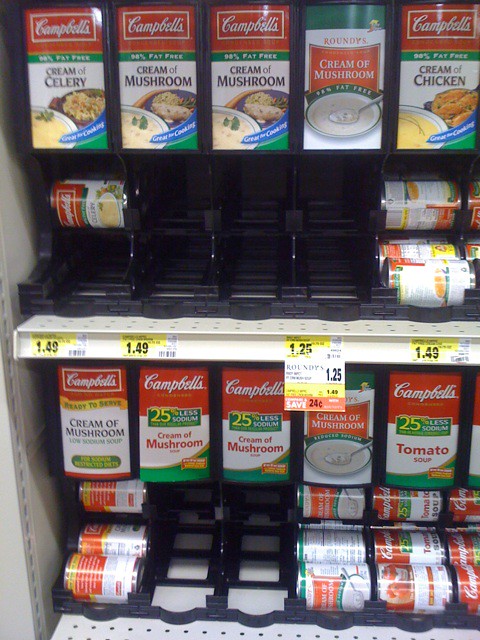This close-up image captures a supermarket shelf in the soup aisle, specifically showcasing an array of Campbell's brand soups. The shelf, constructed from white material, features a sophisticated rack system where black plastic containers hold the soup cans sideways, allowing them to roll forward for easy access as one is taken. In the topmost rack, boxed soups are prominently displayed, including Campbell's Cream of Mushroom, Campbell's Cream of Chicken, and a smaller, different brand's Cream of Mushroom. The soups continue on the lower racks with Campbell's Cream of Celery, Tomato, and various reduced-fat options. The tins are stored beneath the boxed soups in dispenser units. Yellow price labels with black writing and a barcode indicate a price of $1.49 for Campbell's soups, with some items on sale for $1.25. Some shelves appear to be partially emptied, underscoring the popularity of certain varieties.